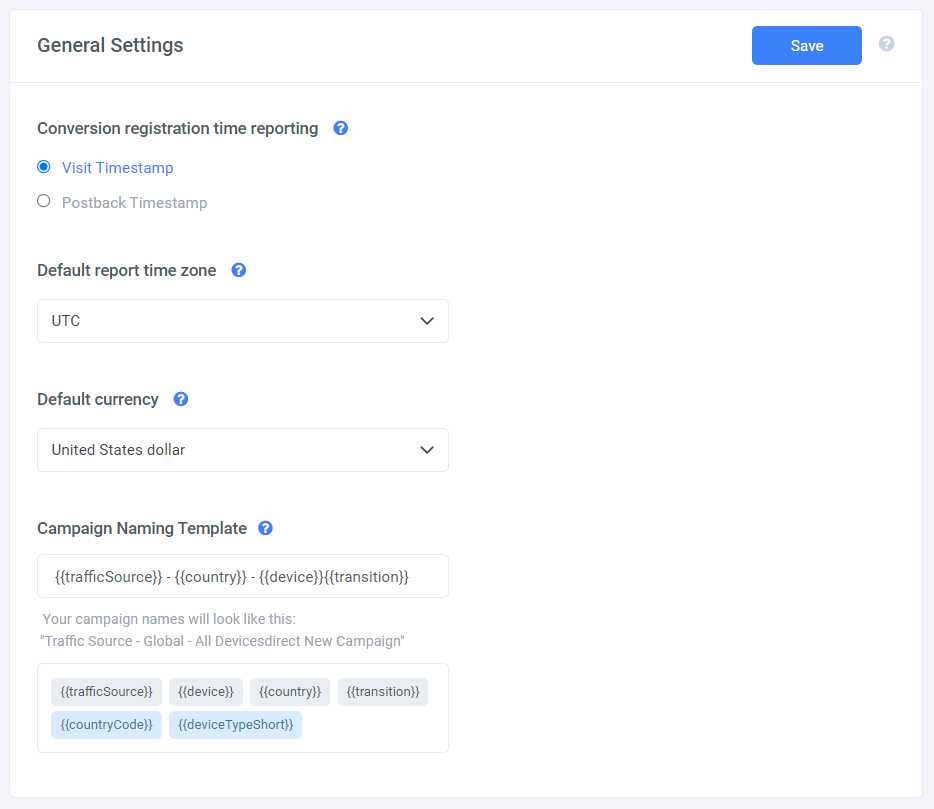The screenshot depicts a computer interface showcasing a detailed view of the 'General Settings' section of an application. The interface is framed by a gray border and features a top bar with the title 'General Settings' in black font. To the right of this title, there's a prominent blue 'Save' button, and next to it, a gray question mark button for additional help.

Below the top bar, the main section is divided into various settings categories:

1. **Conversion Registration Time Reporting**: This section includes a blue, clickable question mark for more information. Users have two options: 'Visit Timestamp' or 'Post Fax Timestamp,' with 'Visit Timestamp' currently selected.
 
2. **Default Report Time Zone**: Accompanied by a blue question mark for assistance, this setting has a dropdown menu where 'UTC' has been selected.

3. **Default Currency**: This setting also features a dropdown menu, currently set to 'U.S. Dollar.'

4. **Campaign Naming Template**: For campaign names, the template requires the format to include traffic source, country, device, and transition within parentheses. An example provided is: 'traffic source (global) (all devices) (direct) (new campaign).'

Additionally, at the bottom of each section, there are interactive buttons to further configure these settings.